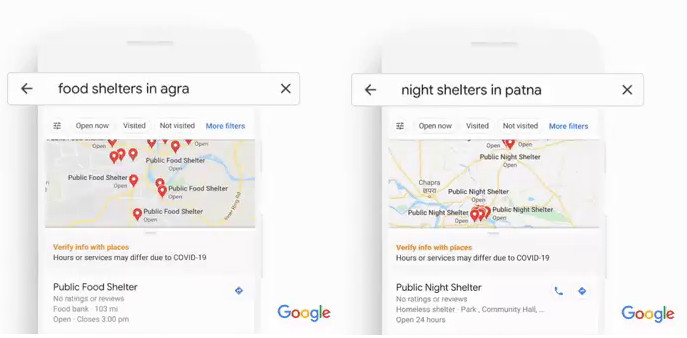The image displays two screenshots from a navigation or mapping application. The first screenshot shows a search result page for "food shelters in Agra," while the second is for "night shelters in Patna." 

In the "food shelters in Agra" screenshot:
- At the top, there is a black back arrow on the left and an X symbol on the right.
- Below these, options for "Open Now," "Visited," "Not Visited," and "More Filters," the latter being in blue font, are available.
- The screen is associated with a map service named "JoJoMap." 
- A yellow notification advises users to "Verify info with places. Hours or services may differ due to COVID-19."
- Listed below is a public food shelter with no ratings or network connection, identified as a food bank.
- The location is 103 miles away and is open until 3:00 p.m.

In the "night shelters in Patna" screenshot:
- It mirrors the layout of the first screenshot with a back arrow to the left and an X to the right.
- Users are again notified to "Verify info with places. Hours or service may vary due to COVID-19."
- The main search result is a public night shelter, categorized as a homeless shelter, park, or community hall, and available 24 hours.
- Icons displayed include a phone and a triangle.
- To the extreme right, the Google logo is visible with its characteristic colors of red, green, blue, and yellow.

Both screenshots emphasize the importance of verifying information with the respective places due to potential changes in hours or services due to COVID-19.